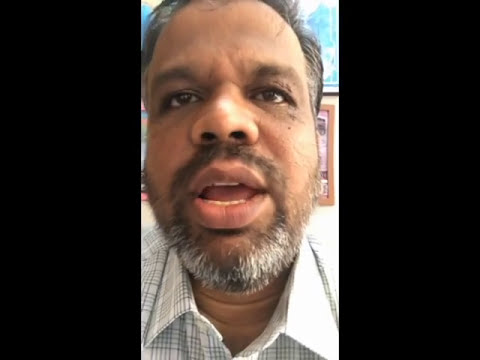This is a close-up photograph of a middle-aged man, possibly of Indian descent, who appears to be in the midst of speaking. He is wearing a neat white button-up collared shirt with a pattern of black lines and squares. The man's short, dark hair is interspersed with gray, and he sports a black and gray goatee and mustache. His light brown skin and expressive face, captured clearly in the image, shows his mouth open, revealing part of his teeth and tongue, as if he is caught mid-sentence. This suggests he might be delivering a lecture, speaking for social media, or engaged in some form of public speaking. The background is obscured by his head, but there is a hint of blue artwork and another partially visible frame, neither of which can be clearly identified due to his proximity to the camera. The image is primarily focused on his face, emphasizing his expressive features and the moment of speech.